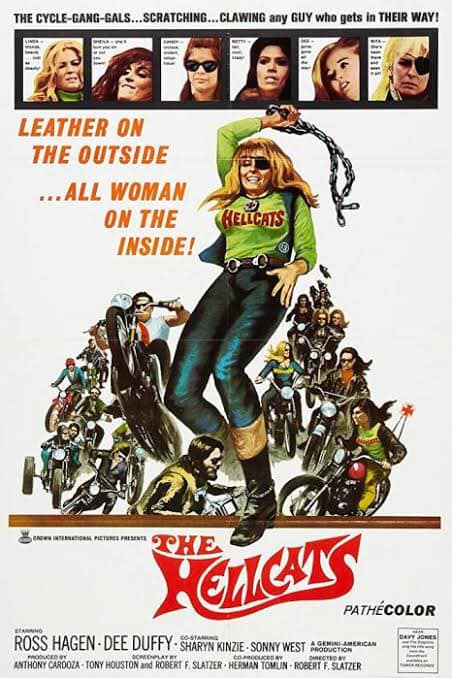This tall rectangular movie poster features a vintage design likely from the 1960s or 1970s, characterized by its aged and illustrative artwork. The background is a light gray color, enhancing the boldness of the elements on the poster. At the top, in bold black capital letters, it reads: “THE CYCLE GANG GALS… SCRATCHING… CLAWING ANY GUY WHO GETS IN THEIR WAY!” Directly below this tagline is a sequence of six square images displaying various women with different facial expressions and hair colors, each bordered by thick black lines. The smaller text adjoining their faces is indiscernible due to its diminutive size.

Beneath these images, in bright orange, italicized capital letters, another tagline proclaims: “LEATHER ON THE OUTSIDE… ALL WOMAN ON THE INSIDE.” Central to the poster is a striking illustration of a woman with blonde hair and bangs, wearing an eye patch. She is clad in a long-sleeve green shirt emblazoned with the word “HELLCATS” in bright red letters, along with blue jeans and black boots. She is depicted swinging a chain above her head with her right arm, with scenes of people riding motorcycles situated behind her, amplifying the action-oriented theme.

The title of the movie, “THE HELLCATS,” is prominently displayed beneath this charging figure. Below the title, the poster lists the film's stars: Ross Hagen, Dee Duffy, co-starring Sharon Kinsey and Sonny West. Additional production credits appear at the bottom alongside a note about the film being in Pathécolor, wrapped up with more unreadable text inside a small box.